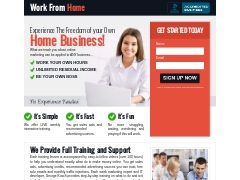This image showcases a low-quality, pixelated webpage. The overall resolution is poor, making much of the text difficult to decipher. 

In the top left corner, there is a legible heading that reads "Work from Home." On the top right, there is a blue button with white text, although the text is too blurry to be read clearly. Below this header, on the left side of the page, there is a slogan that states, "Experience the freedom of your own home business!" Unfortunately, the smaller text beneath this slogan is too blurry to read.

Further down, three check mark icons are visible, each followed by accompanying text which is also unreadable due to its small, fuzzy presentation. 

To the right of this text-heavy section is an image of a smiling woman. She has brown hair that falls to her shoulders, obscuring her ears. Her facial features, including her eyes, nose, and open mouth, can be seen clearly despite the low image quality.